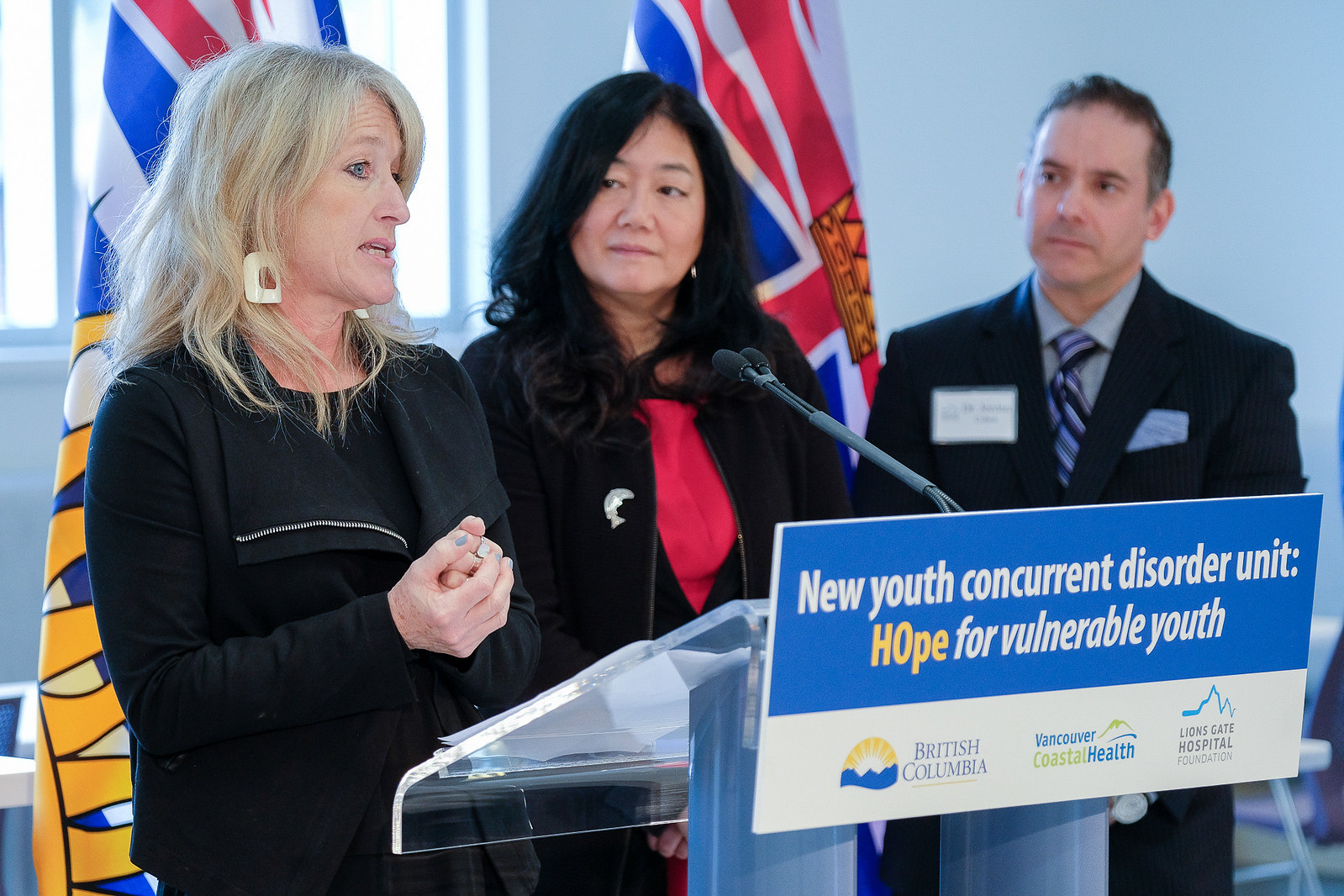The image captures a political press conference set in British Columbia, highlighting the announcement of the "New Youth Concurrent Disorder Unit" signposted with "HOPE for Vulnerable Youth." The speaker at the clear glass podium is a middle-aged woman with long blonde hair, wearing black clothes complemented by distinctive droopy earrings. The podium bears a blue sign with the unit’s name in white and yellow, above the logos of British Columbia, Vancouver Coastal Health, and Lionsgate Hospital Foundation. To her left stands an Asian woman with long black hair, dressed in a red shirt beneath a black jacket, observing the speaker intently. Further to the left is a man in a black suit, equipped with a name tag, a pocket square on his left side, and a striped tie. The backdrop features red, white, and yellow flags alongside a white wall, epitomizing the formal and significant nature of the event.